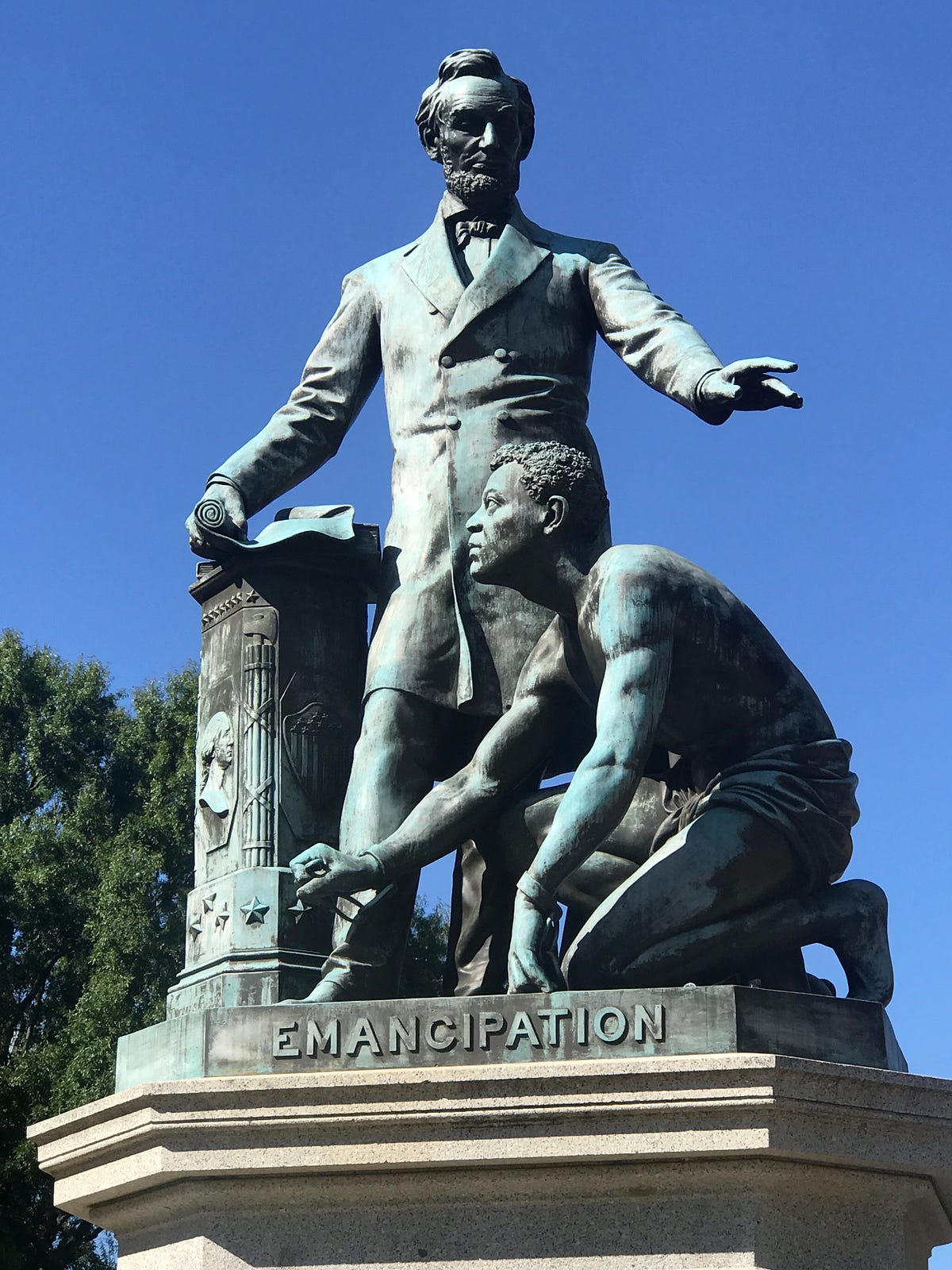The image features a patinated, copper statue of Abraham Lincoln adorned in his traditional long, buttoned blazer. He stands with his left arm outstretched above a newly freed black man kneeling on one knee, dressed only in a loincloth with visible shackles on his wrists and holding his own chain. Lincoln holds a rolled-up document in his right hand, which rests against a three-foot podium. The podium is intricately carved with the figurehead of George Washington and an aged representation of the American flag, complete with stars at its base. The pediment under the figures proudly displays the word "Emancipation" in raised letters. The statue is situated outdoors, against a backdrop of a bright blue sky with green deciduous trees on either side, suggestive of a park setting.